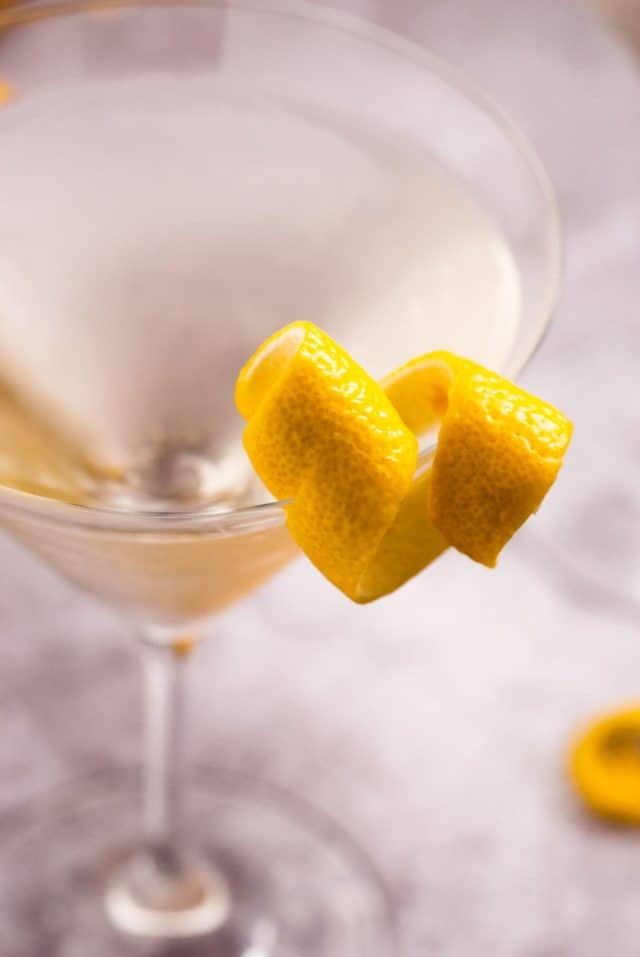The image depicts a close-up shot of a refreshment scene centered on a martini glass filled with a clear to white liquid. The main focus is on the carefully garnished drink, highlighted by a curled ribbon of lemon peel resting gracefully on the glass's rim. The liquid inside the glass exhibits subtle yellow and orange highlights, possibly due to the surrounding lighting. The martini glass has a slender, elongated stem and a broad, circular base, which slightly blurs into the background. It is perched on a table adorned with what appears to be a muted pink and gray tablecloth, although the tablecloth is somewhat blurry and cropped at the edges. The overall ambiance of the photo is soft and inviting, despite the general blur present throughout the image.